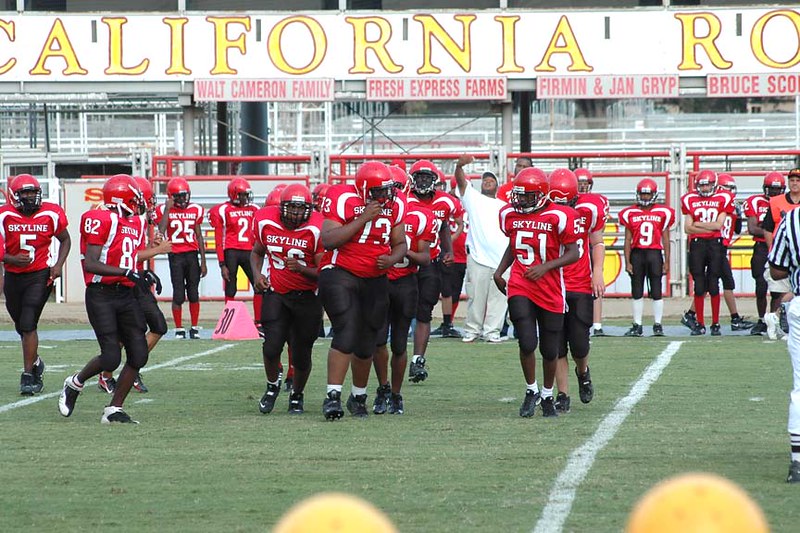The photograph captures a junior football team during a game on a verdant, striped field characterized by short green grass and white yard lines. The players, likely teenage boys, are attired in black pants, black cleats, red jerseys adorned with the word "SKYLINE" in white letters, and red helmets featuring black face cages. Approximately 10 to 15 players are visible on the field, engaging in the game, while additional players and possibly coaches stand along the sideline. Dominating the background, a white banner with yellow letters outlined in red partially reads "California RO," with further sponsors listed below: Walt Cameron Family, Fresh Express Farms, Herman and Jan Grip, and Bruce Spill, the latter being cut off. Metal bleachers and a referee can also be seen in the scene, hinting at a lively, organized sporting event.